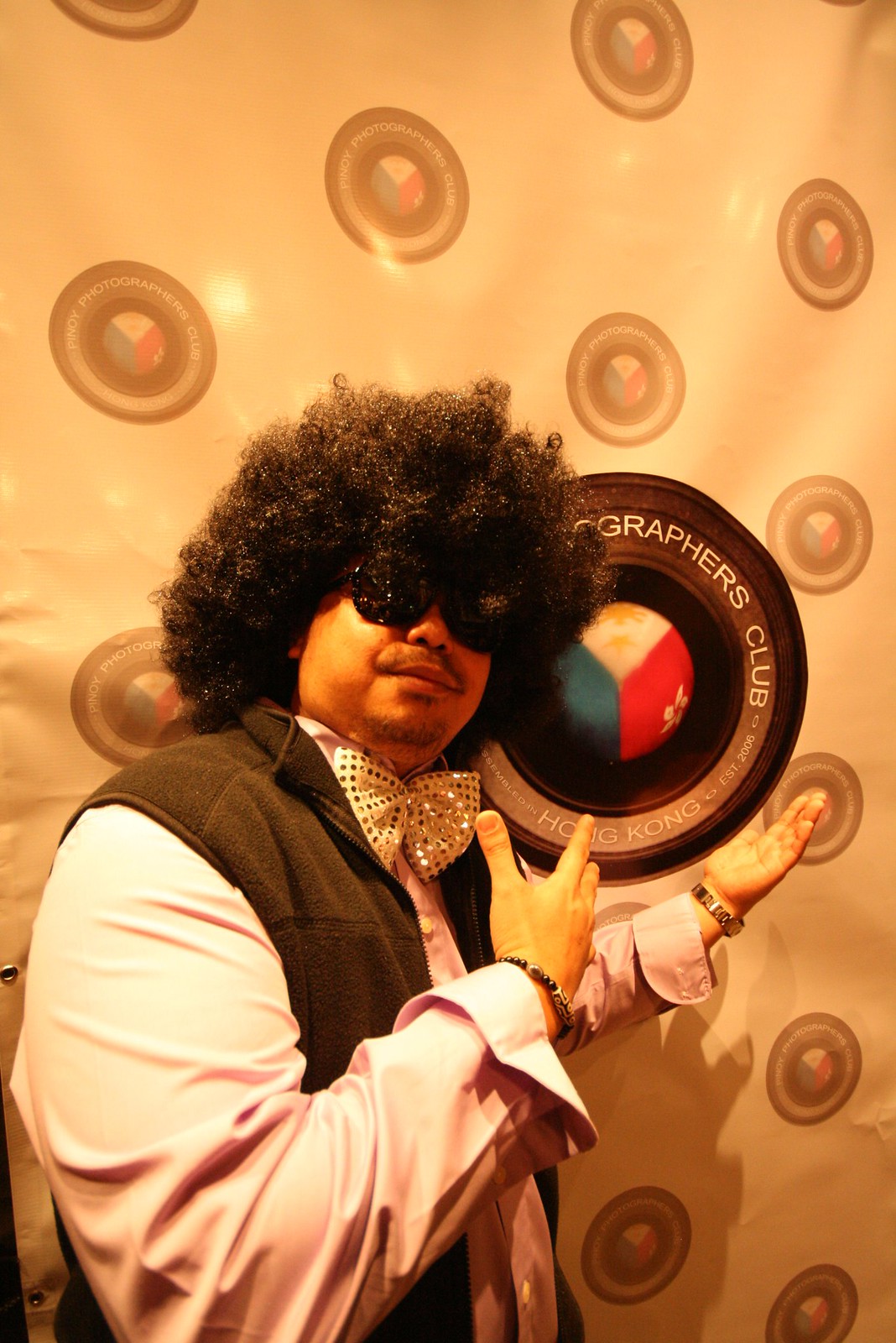In this color photograph, a black male stands confidently in front of a white banner with a patterned design featuring smaller circles and a larger central circle with the text "Photographers Club" surrounding a black camera ring and an emblem resembling an upside-down peace sign with red on the right, blue on the left, and a white triangular slice at the top. The man, wearing a large afro wig and black sunglasses, is dressed in a long-sleeved pink collared dress shirt paired with a gray vest, and a sparkling silver bow tie. He sports a thin mustache and a thin, well-trimmed goatee. On his left wrist, he wears a watch, while a bracelet adorns his right wrist. His body is turned to the side, but his face is directed towards the camera, capturing his animated pose. His left hand points towards the "Photographers Club" sign behind him, and his right hand is slightly raised beneath it, as if presenting the logo.